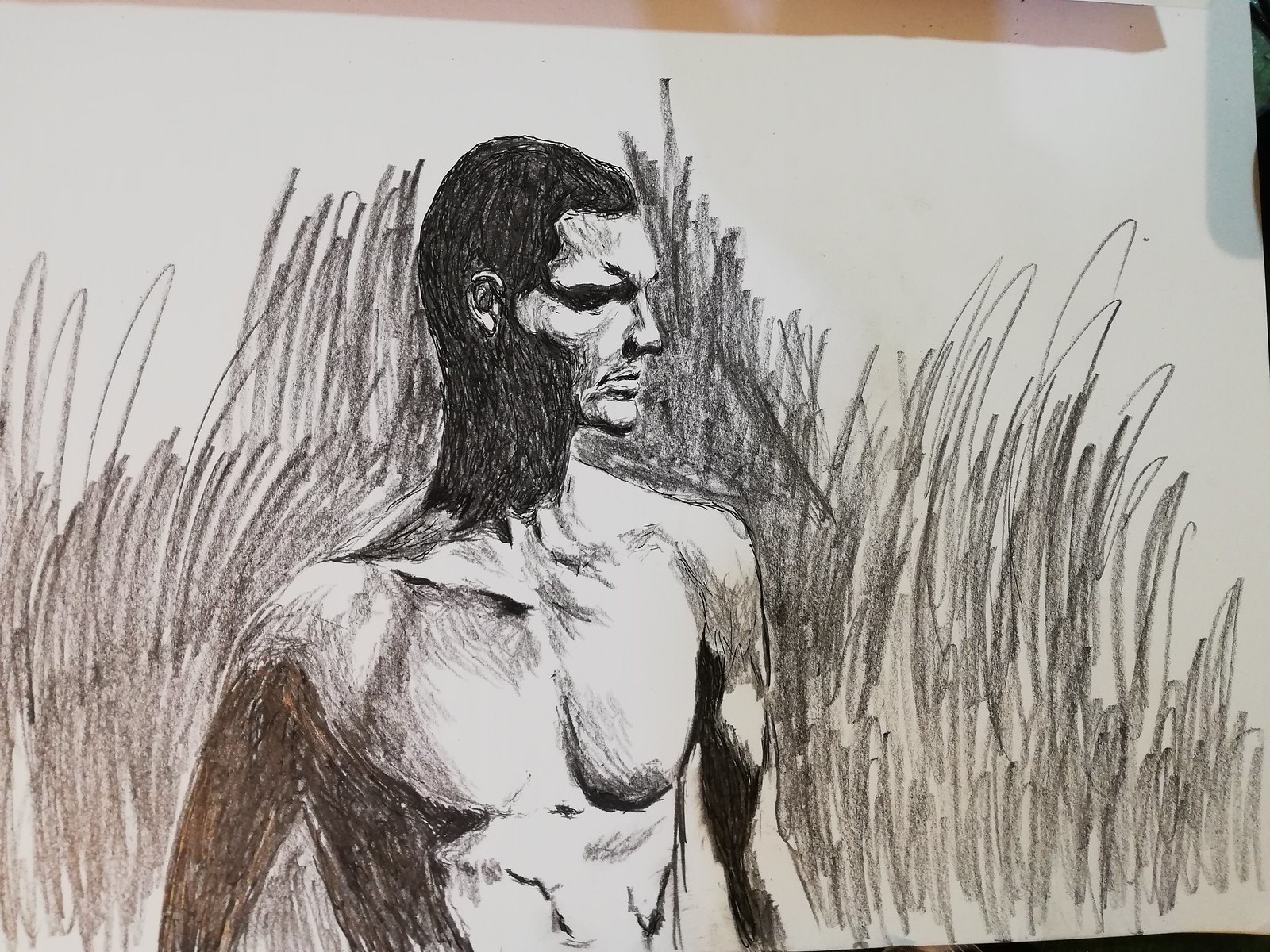This detailed black and white sketch, rendered on standard white paper—possibly from a sketchbook or even just printer paper—depicts a shirtless man from the ribcage up. The artist, using what appears to be charcoal or a sketch pencil, has intricately captured the man’s short dark hair and strong features. His facial expression conveys a sense of sternness or deep concentration, adding a layer of intensity to the portrait. The background is filled with a series of lines and scribbles, which could either represent tall grass or serve as an artistic choice to add texture and depth to the drawing. The man's slightly muscular build and the intricate detailing further emphasize the skill and effort put into this grayscale composition.